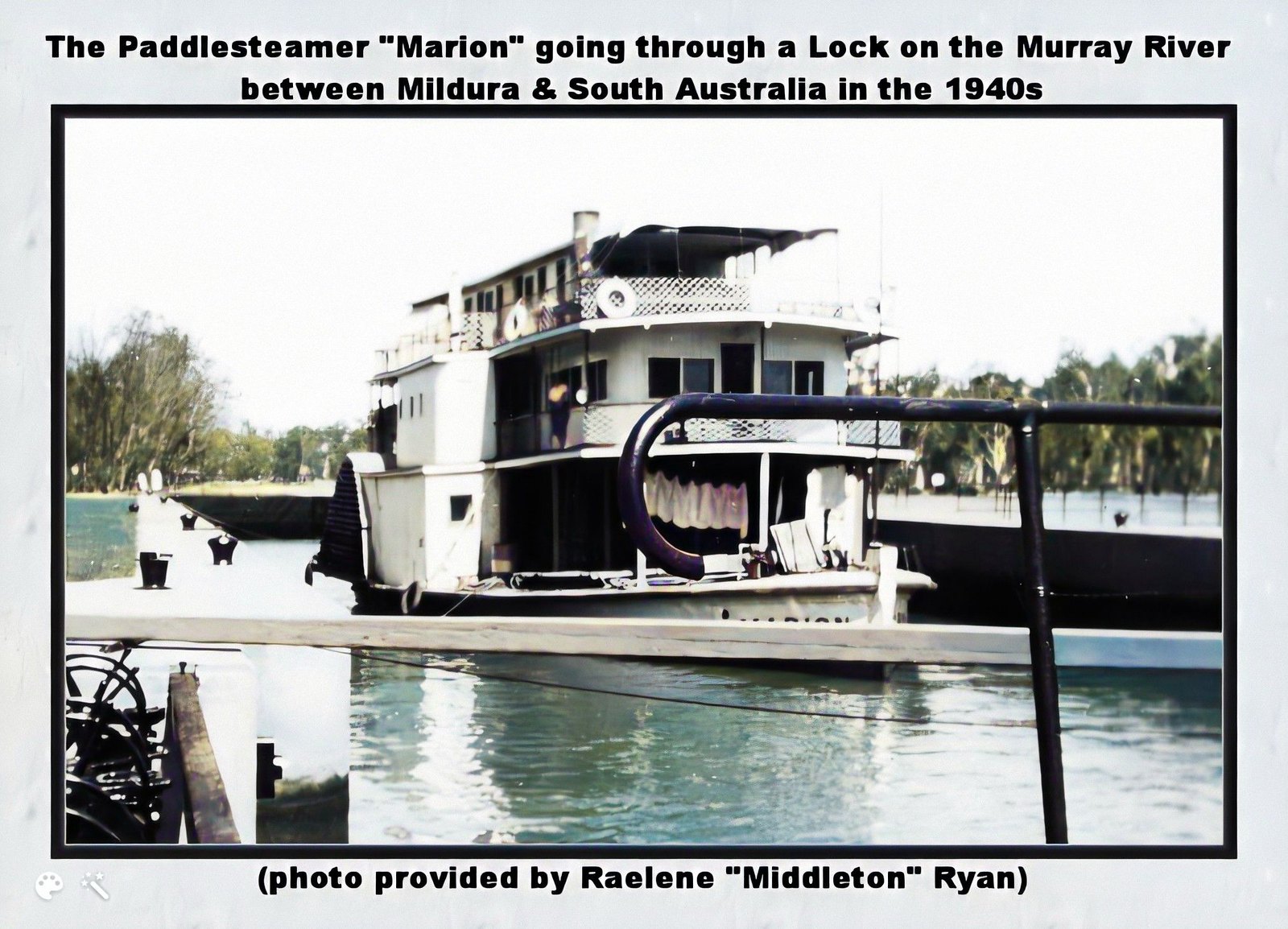The image captures a detailed photograph of the paddle steamer Marion navigating through a lock on the Murray River, located between Mildura and South Australia, during the 1940s. The boat, prominently white in color, features three levels and is seen floating on the bluish-green water of the river. The scenery includes various structures and fencing along the riverbanks, as well as an obstructive wooden and metal fence in the foreground, enhancing the depth of the image. In the background, lush greenery and trees are set against a white sky. A noteworthy detail includes a white pole extending across the water, and a black piece of machinery is visible in the lower left corner. Bordering the photograph is a thin black frame surrounded by a thicker light blue frame. The top border of the image contains the text: "The paddle steamer Marion going through a lock on the Murray River between Mildura and South Australia in the 1940s." The bottom border reads: "Photo provided by Raylene Middleton and Ryan."